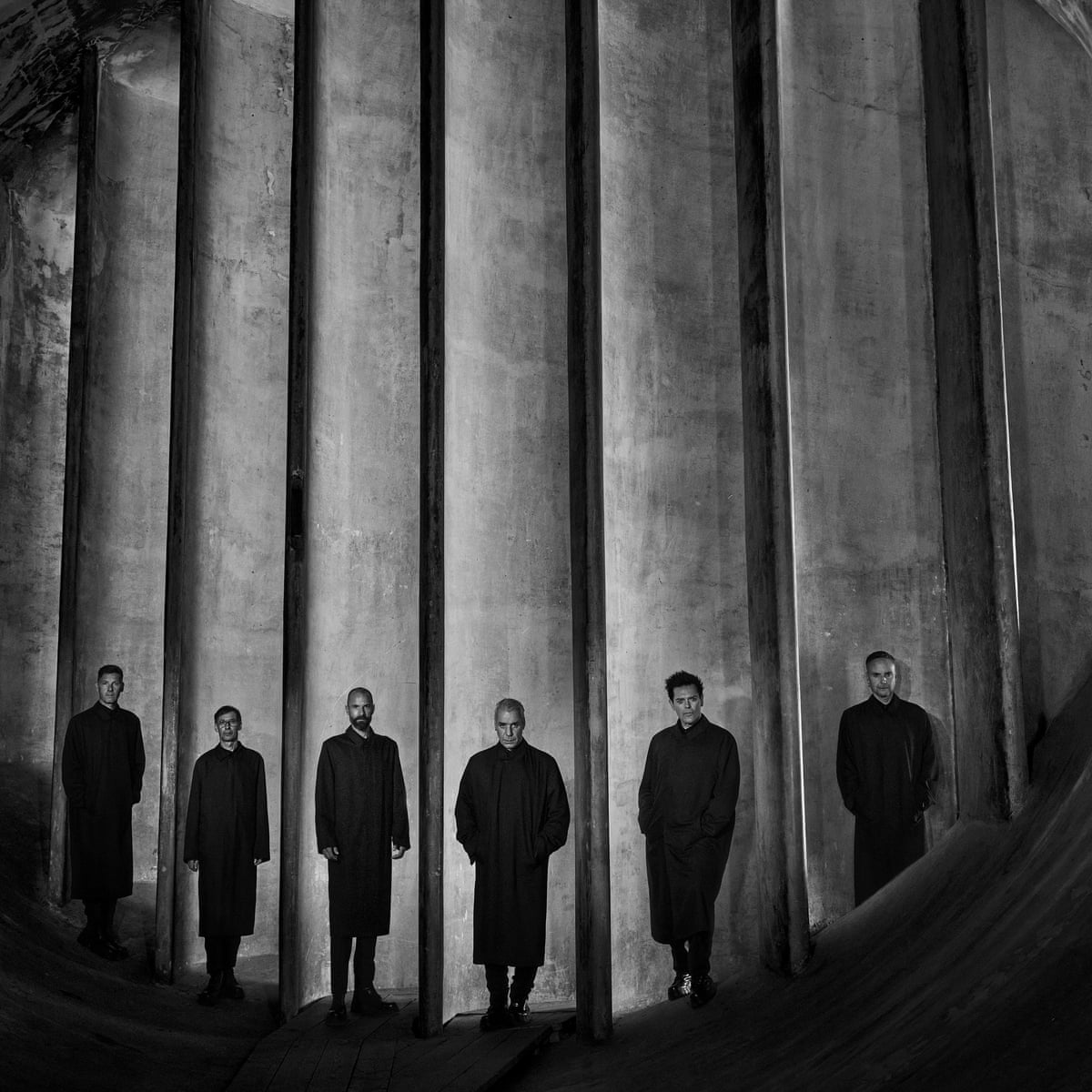This vertically rectangular black and white photograph features six men standing side by side in individual cubby-like enclosures. Each man wears a long black trench coat, paired with black pants and black shoes or boots, creating a uniform appearance. The men, all appearing to be under the age of 40 with short hair, stand against a backdrop of tall, vertical columns that form a seemingly endless wall, extending upwards at least 20 feet, disappearing out of the frame. The columns have a grayish tint, adding to the monochrome aesthetic of the image. The bottom portion of the walls forms a curved wooden semicircle that borders each man's platform. The lower part of the image is solid black, enhancing the distinct separation of each individual while emphasizing the unity of the group.